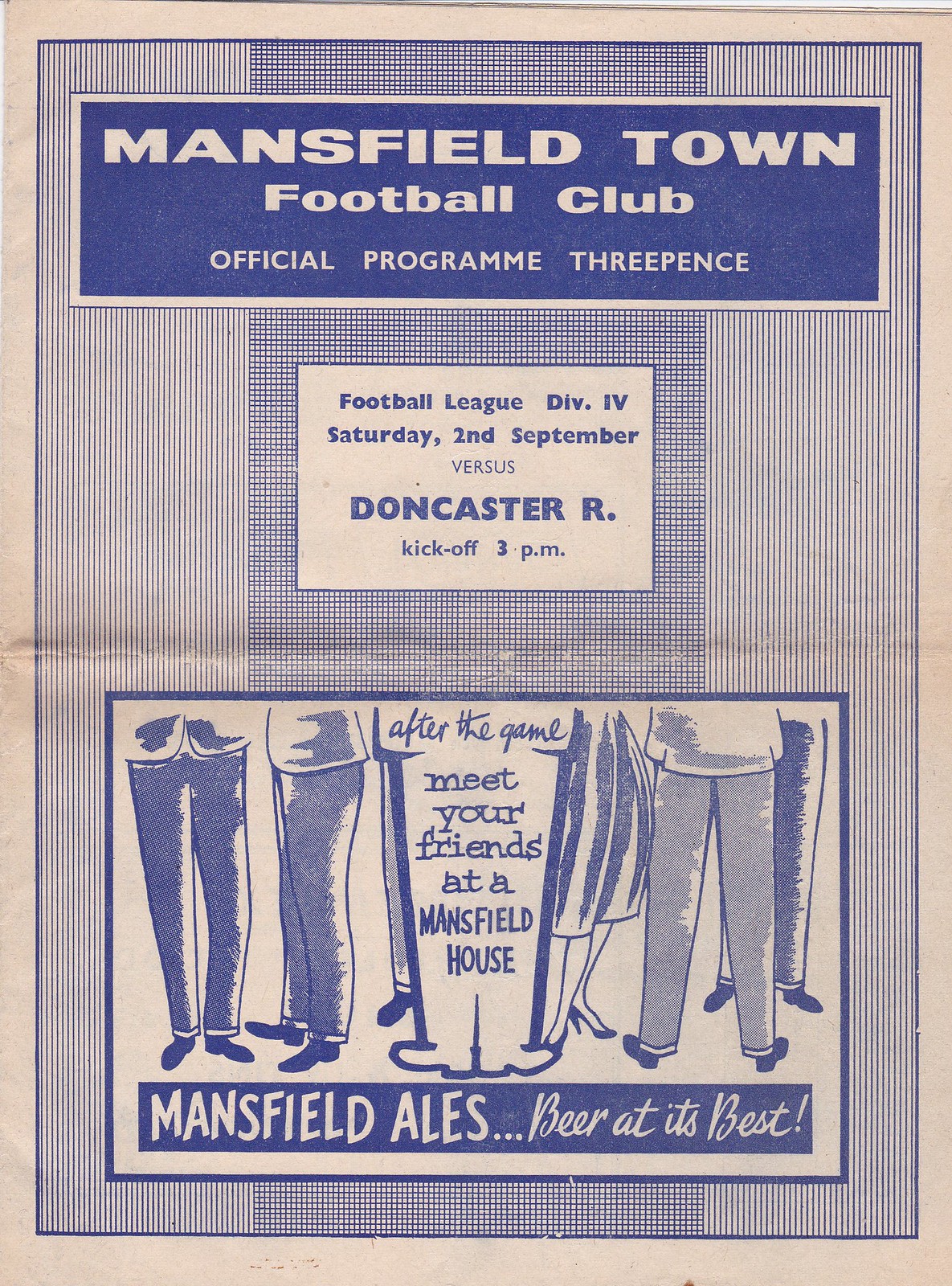This image features a vintage program from the Mansfield Town Football Club, priced at three-pence, displayed in a worn, folded state, adding to its historical charm. Positioned prominently at the top, within a blue box with white text, reads "Mansfield Town Football Club Official Program, Three-Pence." Below this, another box, resembling the slightly whiter background hue of aged newspaper, details the event: "Football League Division 4, Saturday, 2nd September versus Doncaster R, kickoff 3 p.m." The program is characterized by its blue newsprint with a fading, off-white, almost tannish background. Thin vertical lines are present on the left and right edges, while the center features a crosshatch pattern, creating a visually distinct section. At the bottom, an advertisement displays a drawing of people in early 1960s attire, with men in trousers and one woman in a knee-length dress, showcasing only their legs up to their belly buttons in a cartoonish style. This ad invites fans to "Meet your friends at the Mansfield House" and promotes "Mansfield Ales, beer at its best," capturing the essence of the era with its illustrative flair.